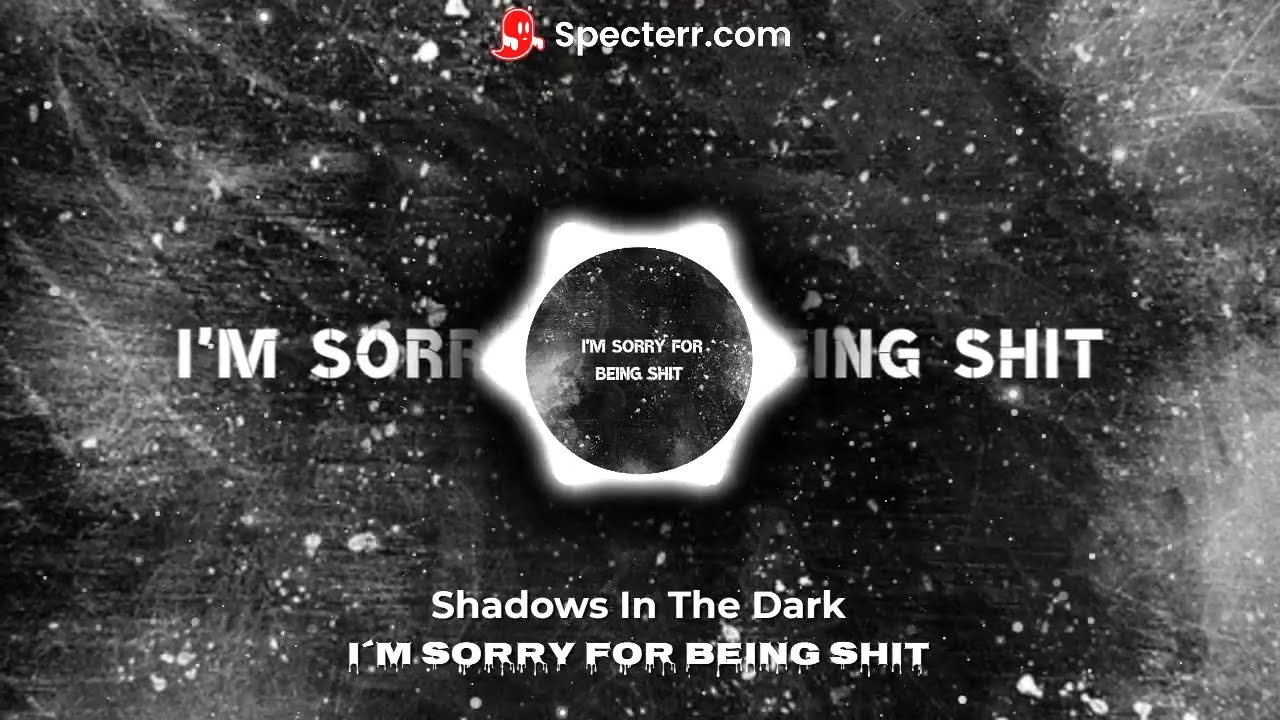The image has a sci-fi, space-like appearance with a rough, grayscale background resembling a worn chalkboard or outer space filled with white dots and nebula-like clouds, giving the impression of a winter storm at night. At the top center, there is a small red ghost with white arms, oval eyes, and a white smile, next to which "Specter.com" is written in white text with an unconventional spelling of S-P-E-C-T-E-R-R. Central to the image is a circle, resembling a planet, surrounded by a glowing six-pointed star. Within this circle, the phrase "I'm sorry for being shit" is prominently displayed in white, while fragmented text "I'm sori...eeing shit" can be seen partly obscured behind the star. Below this central motif, the text "Shadows in the Dark, I'm sorry for being shit" is written in white, with a font that depicts dripping blood, though the drops are white.